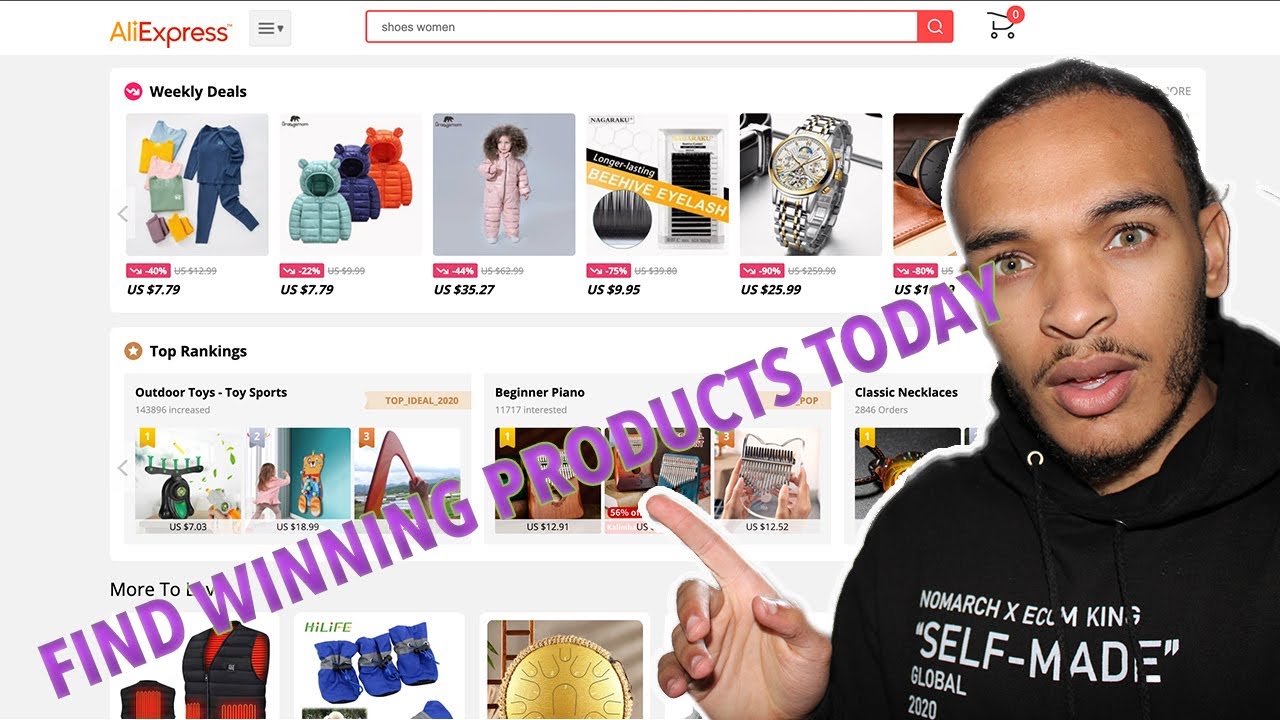In the image, there is a digitally edited thumbnail designed as an eye-catching advertisement. The background prominently features the AliExpress website, characterized by a light gray backdrop displaying the weekly deals, top rankings, and various product categories like baby coats and watches. Layered atop this backdrop, a man is photoshopped onto the right side of the image. He appears to be of Middle Eastern descent, with greenish-brown eyes, a mustache, and facial hair, and black hair. He is dressed in a black sweatshirt adorned with white text reading "No March X Ecom King Self-Made Global 2020."

The man is captured in a dynamic pose, pointing towards a bold, purple text that spans from the bottom left to the top right of the screen, proclaiming, "Find Winning Products Today." This edited text is a clear and inviting call-to-action, aimed at attracting viewers to discover highly recommended products on AliExpress. The man's gesture and the prominent text work in harmony to underscore the call-to-action. 

Additional elements of the AliExpress interface, such as the white boxes showcasing items and a red-outlined search bar at the top, are visible in the background, reinforcing the theme of an online shopping guide.